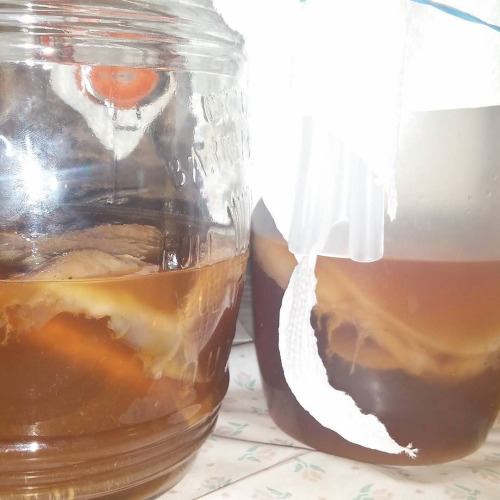In an extremely overexposed photograph taken under intense sunlight, a blurry image shows two glass containers resting on a light-colored counter. The container on the left resembles a large glass jug with a glass cap, partially filled with a brown, tea-colored liquid. Floating within the liquid are cloudy, uneven particles. A red spot, possibly a reflection or a glare, appears on the upper part of the jug, resembling an eye but definitively not an eye. On the right side, another glass container—marked by white irregularities or artifacts likely caused by photocopying or glare—holds a similar tea-colored substance. A citrus-colored label descends into this rightward jar, further adding to the image's obscurity. The overall photograph is notably very, very blurry, making the precise identification of these items challenging.